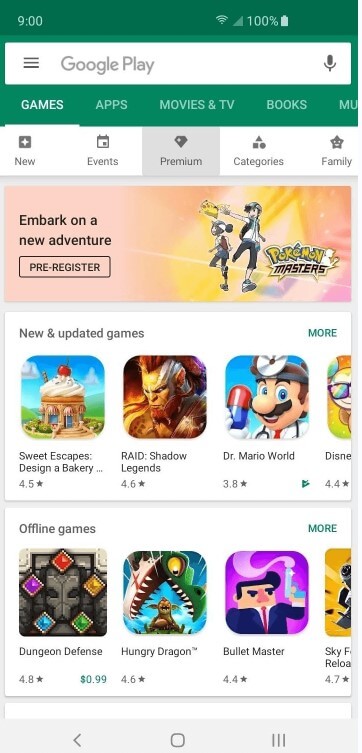This image is a screenshot taken in portrait mode of a mobile device displaying the Google Play Store interface. The topmost section features a green background with three rows. On the upper left, the time is shown as 9:00, while the upper right displays a fully charged battery icon at 100%.

Beneath this, there is a search bar labeled "Google Play," directly under which are tabs for "Games," "Apps," "Movies & TV," "Books," and a selection option for more categories. The "Games" tab is currently highlighted.

The next row, set against a white background, lists navigation options: "New," "Events," "Premium," "Categories," and "Family," with "Premium" being highlighted in gray.

Following this, there is a large banner image spanning the full width of the screen, showcasing "Pokémon Masters." The right side of the banner features animated characters, including two young individuals and a yellow creature resembling a plush toy. On the left, the text reads "Embark on a new adventure," accompanied by a "Pre-register" button.

Below this banner, a white section lists "New & Updated Games," with a green "More" button in the upper right corner. Visible in this section are four game titles: "Sweet Escapes: Design a Bakery," "Raid: Shadow Legends," "Dr. Mario World," and a game beginning with "Disney." Each game includes its respective ratings.

Another white section follows, labeled "Offline Games," displaying titles such as "Dungeon Defense," "Hungry Dragon," and "Bullet Masters," along with an option to view more games.